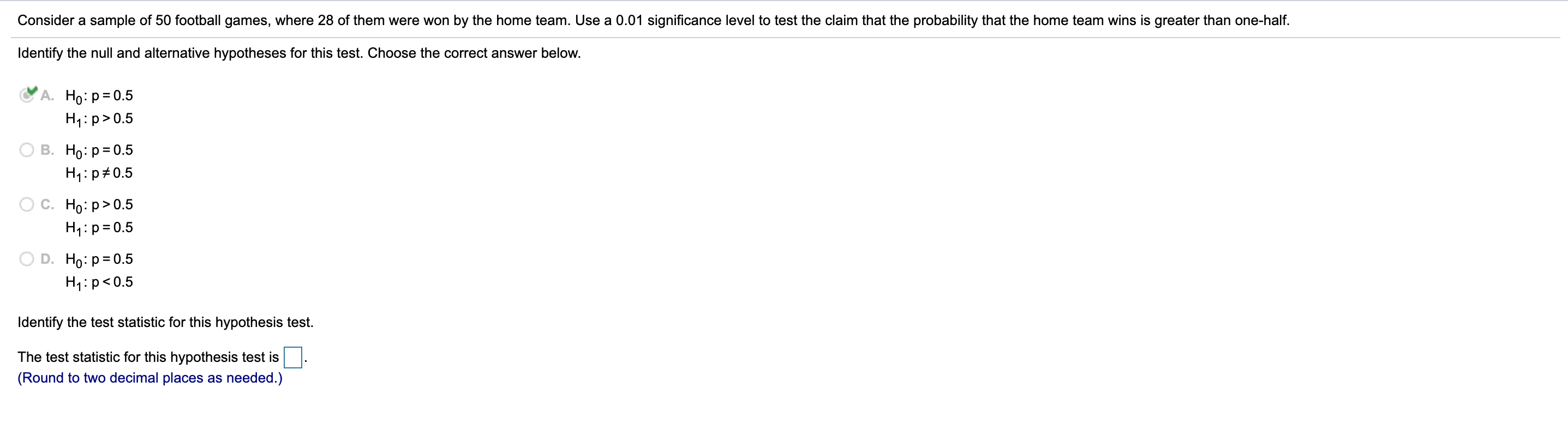The image depicts a test question presented in black text against a plain white background. The text is framed by thin gray lines at the top and bottom for emphasis. The question reads: "Consider a sample of 50 football games where 28 of them were won by the home team. Use a 0.01 significance level to test the claim that the probability that the home team wins is greater than one-half." Following this, there is an instruction that states: "Identify the null and alternative hypotheses for this test. Choose the correct answer below."

Beneath this instruction, there are four options labeled A, B, C, and D, each containing a different set of hypotheses equations. The option labeled "A" has a small circle inside it with a green checkmark over the top, indicating it is the correct choice.

At the bottom of the image, additional text prompts the user to identify the test statistic for the given hypothesis test. It states: "The test statistic for this hypothesis test is," followed by a blank box where the answer should be entered. There is an additional note in blue text that instructs: "Round to two decimal places as needed."